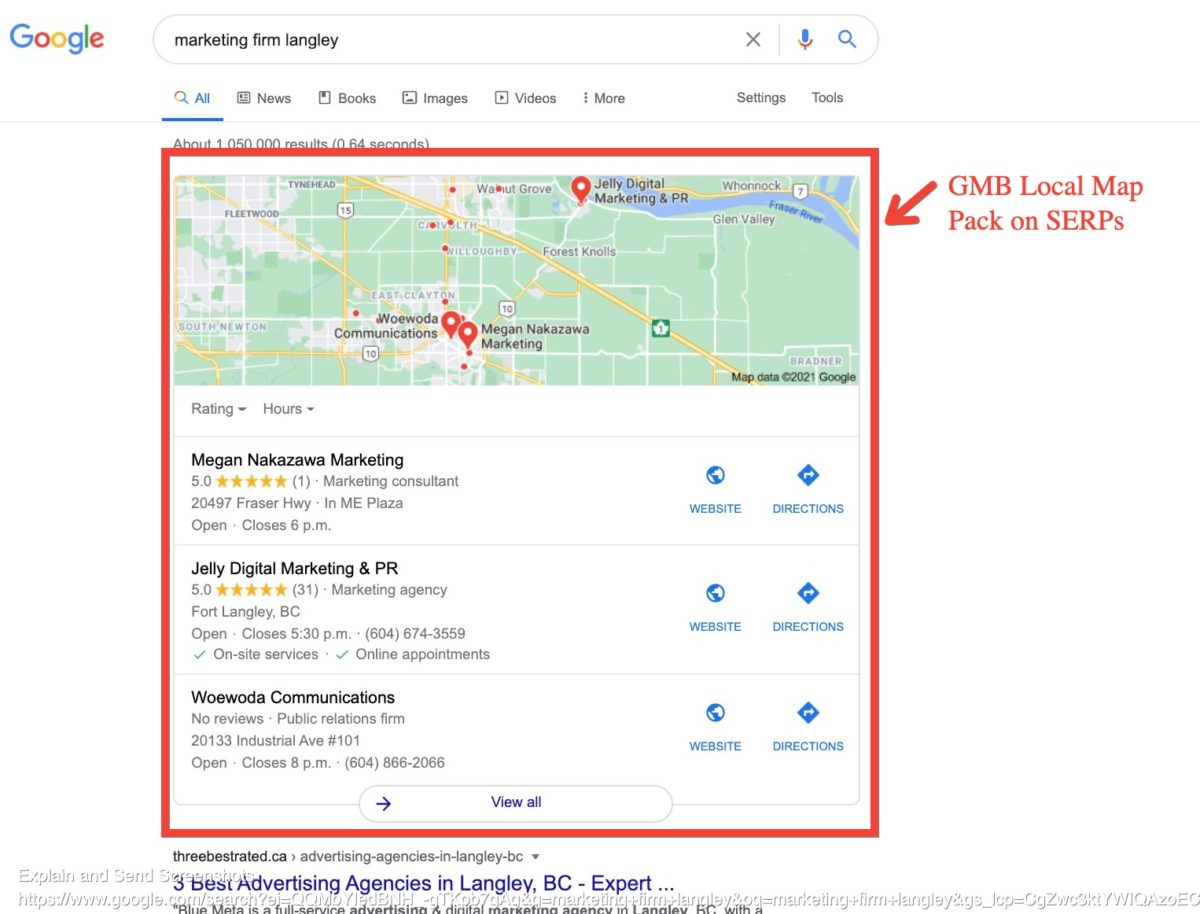**Descriptive Caption:**

The image is a detailed screenshot taken from Google's search results page. In the upper left-hand corner, the Google logo and text are prominently displayed, adjacent to a search bar containing the query "Marketing Firm Langley." The horizontal menu beneath the search bar lists options: All, News, Books, Images, Videos, and More. To the right are the Settings and Tools menus. The 'All' tab is currently selected, revealing approximately 1,050,000 results retrieved in 0.64 seconds.

Highlighted by a red box, the top result in Google's search engine results pages (SERPs) is the JMB Local Map Pack. An arrow points to this box from the upper right-hand side, accompanied by red text labeling it. Within this box, at the top, a map showcases several marketing firms in Langley with precise locations marked. The firms listed include Megan Nakazawa Marketing, Jelly Digital Marketing, NPR, and WoWota Communications, each accompanied by reviews, addresses, and operating hours. On the right side of each listing, there are buttons for visiting the website and obtaining directions, as well as a "View All" button at the bottom for more results.

Outside the red-highlighted box, there is a link to an article titled "Three Best Advertising Agencies in Langley, BC." However, the link is somewhat obscure due to the white text used.